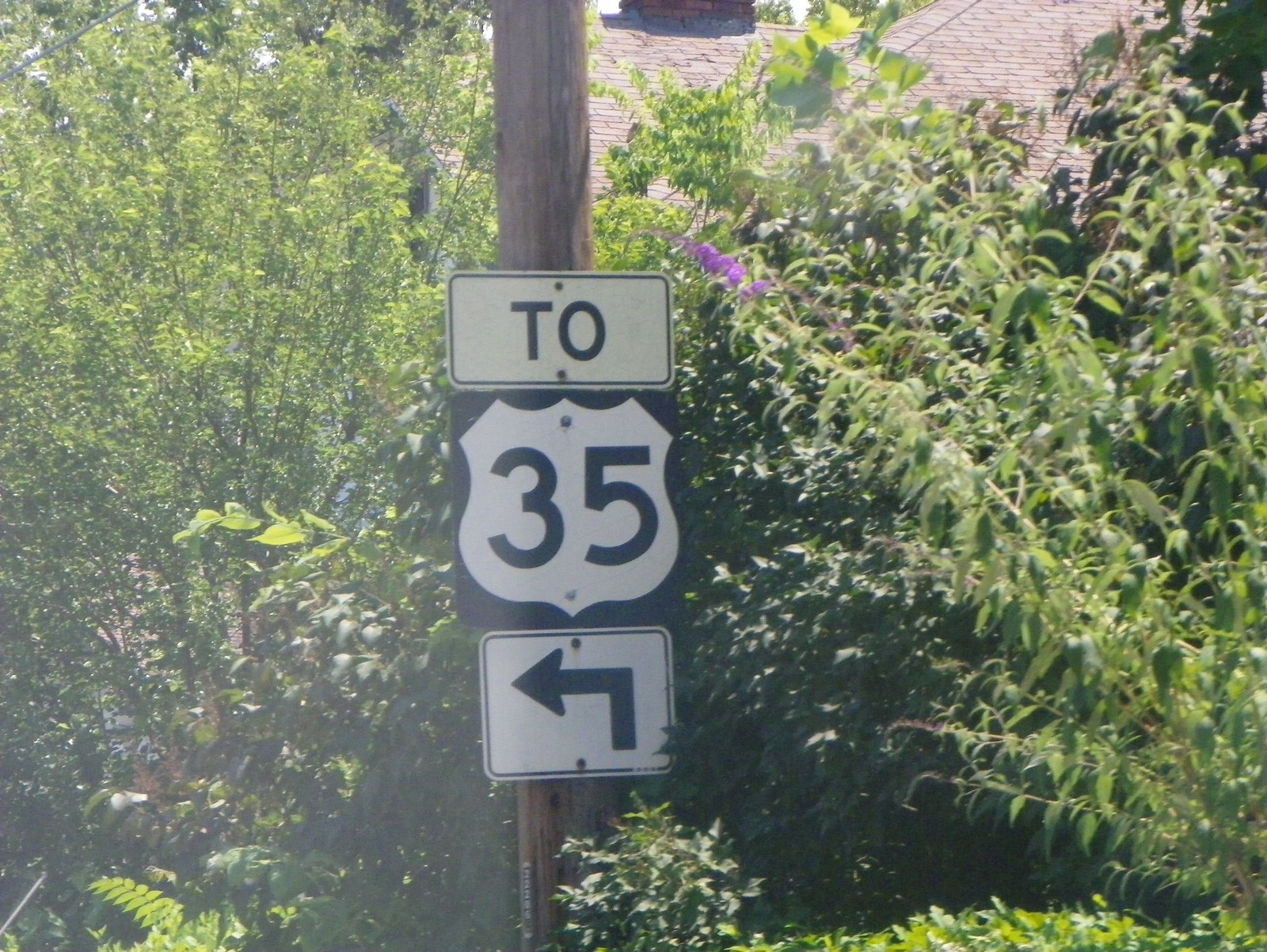This image depicts a wooden utility pole standing tall amidst a backdrop of lush greenery. Firmly affixed to the pole are three distinct signage panels, stacked vertically to form what appears to be a continuous display of information. 

The topmost sign is a horizontally placed rectangle with a white background bordered in black, bearing the letters "TO" in bold, black font. Directly below it, the second panel features a shield-shaped emblem reminiscent of a police badge, also white with a black border, containing the number "35" in prominent black digits. The bottom panel, a square or slightly rectangular sign, showcases a white background with a black border. It has an L-shaped black line with an arrow pointing left at the end of the horizontal segment, directing attention or traffic to the left.

Surrounding the pole, verdant bushes add a touch of nature, interspersed with a small cluster of vibrant purple flowers. In the distance, part of a brown house roof is visible, revealing just the base of a brick chimney. Overhead, the sky appears overcast, with only a sliver visible, leaving the specifics of the weather uncertain.